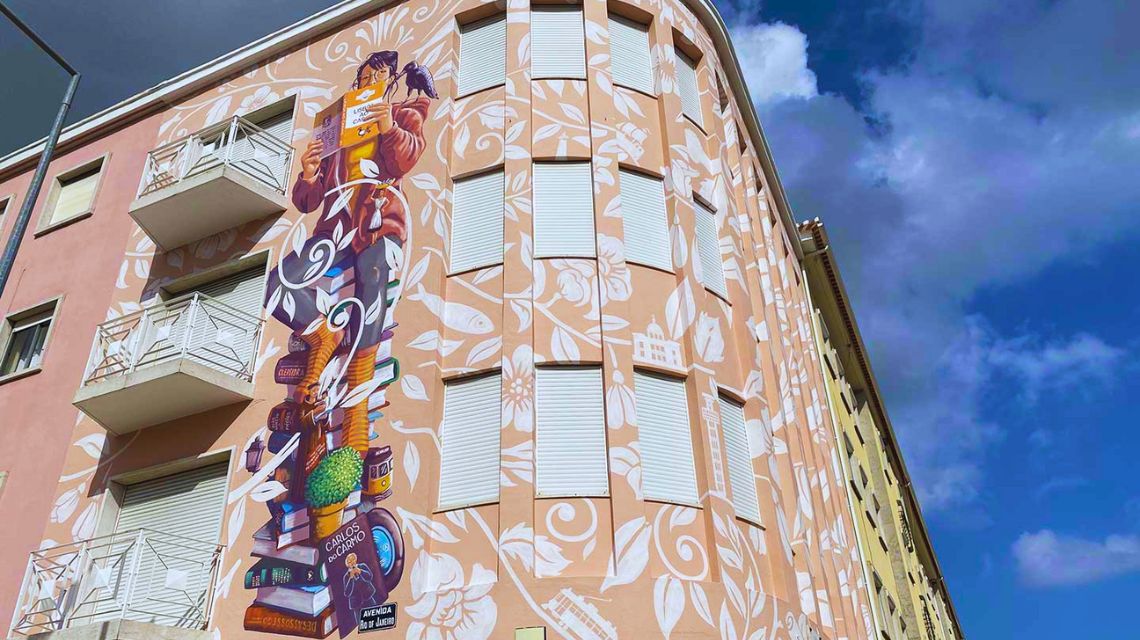The image depicts a multi-story, peach-colored building viewed from below, with a blue sky scattered with both white and darker gray clouds in the background. The building's façade features intricate white etchings of leaves across its surface. A large, colorful mural spans from top to bottom on one side, illustrating a young girl seated on a tall stack of books, holding an orange book, with a raven perched on her shoulder. Surrounding her are additional painted objects such as glasses, fish, and flowers, extending between the windows. The windows, adorned with garage-like gray shutters, are all closed. The building has balconies with similarly closed shutters. The structure curves in a semicircle, forming three rows of four windows each around the bend. A yellow building is attached to it on the side, and there's a red or another peach-colored building adjacent. The roof is lined with a grayish panel, completing the picture of this detailed and art-adorned architectural scene.